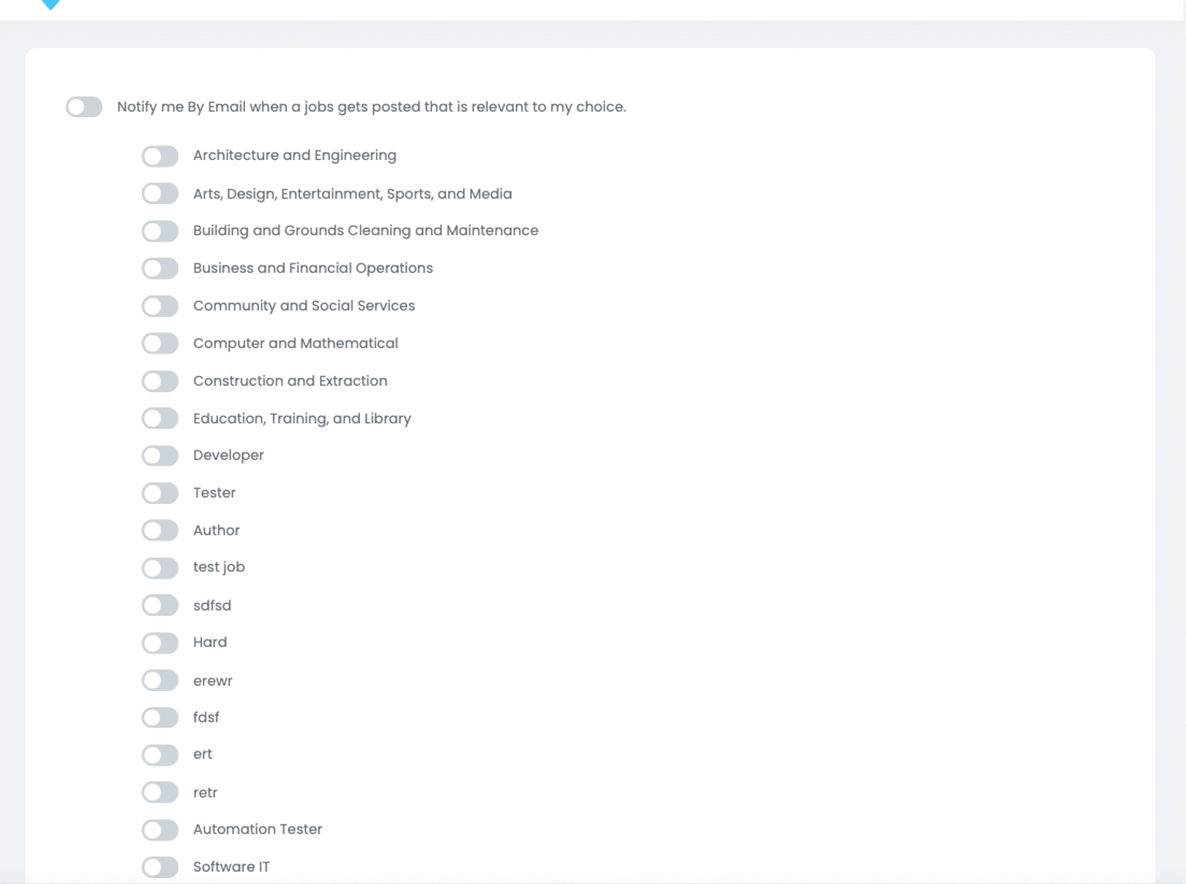The image is a screenshot of an unknown website featuring a set of job notification settings. At the top, there is a notification option that users can toggle on or off. The notification text reads: "Notify me by email when a job gets posted that is relevant to my choice." Below this option is a horizontal scrolling menu for selecting job categories. Users can navigate through the categories using left and right arrow buttons.

The visible job categories on the website are:

1. Architecture and Engineering
2. Art, Design, Entertainment, Sports, and Media
3. Building and Grounds Cleaning and Maintenance
4. Business and Financial Operations
5. Community and Social Services
6. Computer and Mathematics
7. Construction and Extraction
8. Education, Training, and Library

Additional job categories, which seem to include some non-standard or placeholder names, are:

9. Developer
10. Tester
11. Author
12. Test Job
13. FSD
14. Couple of HARD
15. AREWR
16. TDSF
17. ERT
18. RETR
19. Automation (with capital A)
20. Tester (with capital T)
21. Software (with capital I and T)

Each category has a "Select" button next to it, allowing users to choose the type of jobs they want to be notified about.